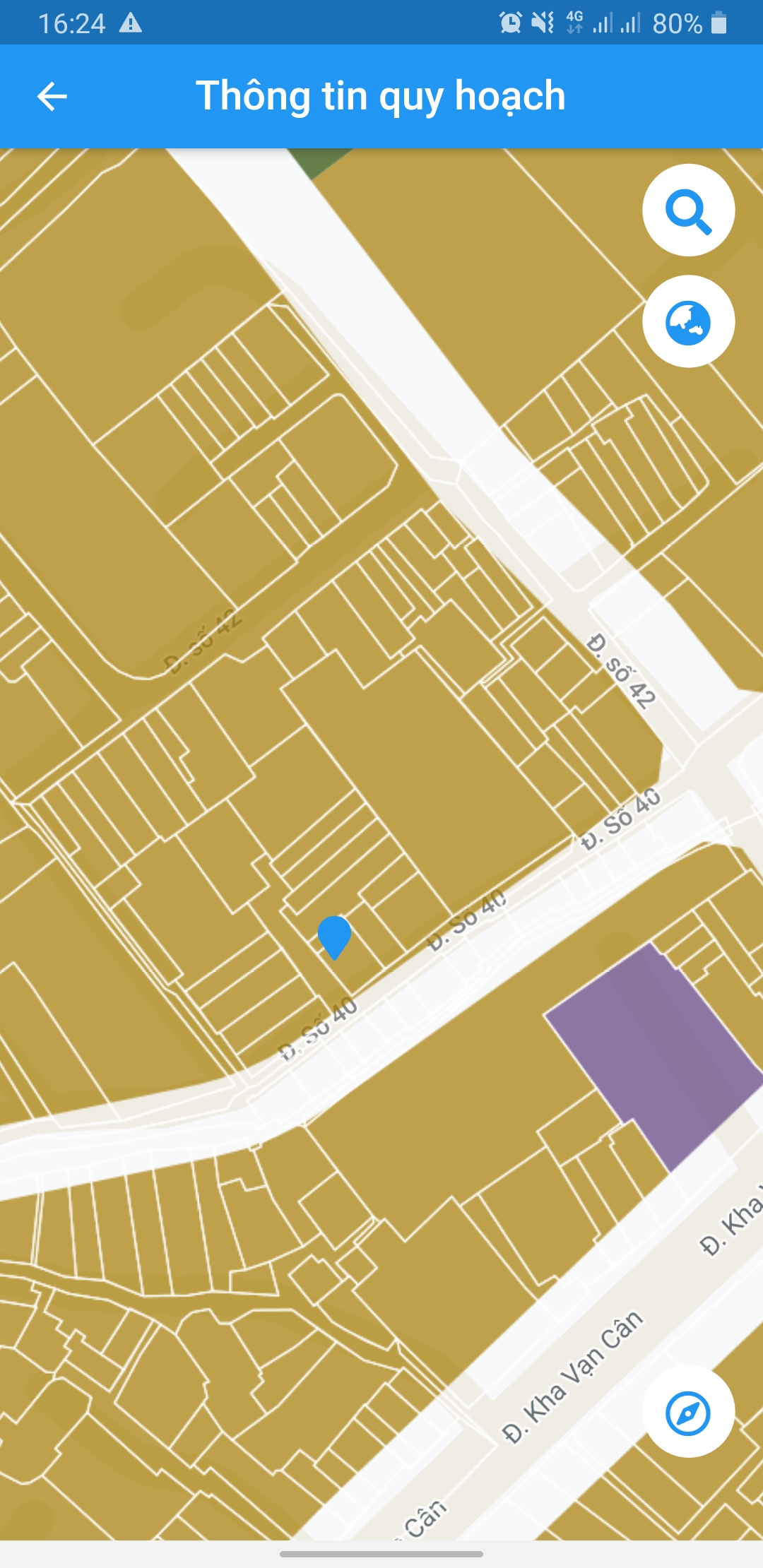The image depicts a screenshot from a mobile phone displaying a map, likely from Google Maps. A blue pinpoint is placed on a specific location on a building along a street that resembles "S O 40." Another larger street, labeled "Kha Vancan," intersects nearby. The map indicates a timestamp of "6:24" in the top corner and shows the phone battery at 80% charged. 

At the top of the screen, there is a blue bar with a back button icon and text that reads "Dong Ting Ki Watch." The bottom right corner features a compass icon, while the top right corner displays a search icon and a Google Earth icon. Notably, the map highlights one structure in purple while the surrounding buildings are colored yellow, emphasizing its distinctiveness.